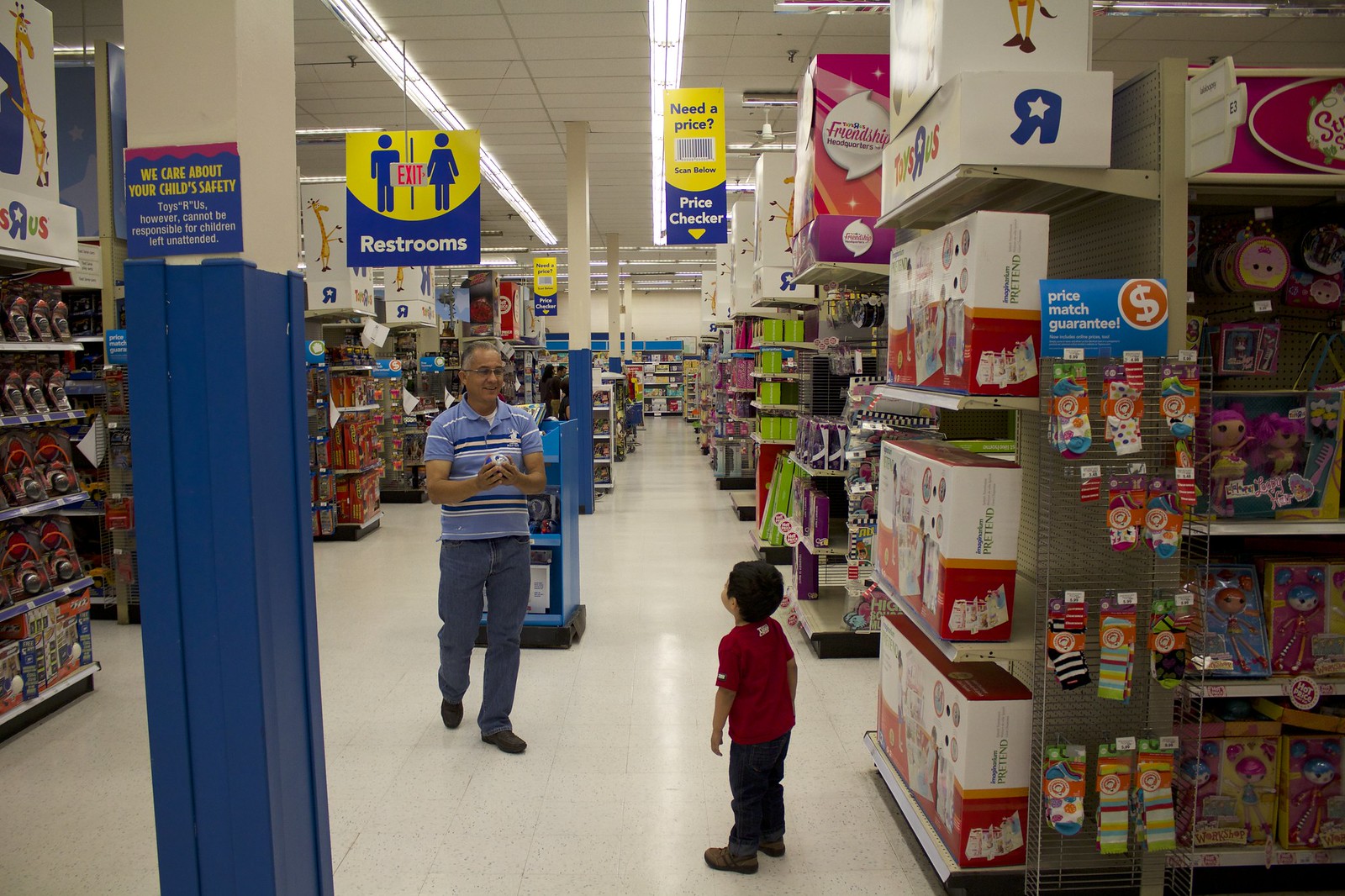This photograph captures a vibrant scene inside a Toys "R" Us store, focusing on a central aisle. In the middle of the image, a man is walking toward a little boy, both facing each other. The man is dressed in a blue striped shirt and blue jeans, while the little boy sports a bright red shirt paired with jeans. Above the man, a vivid yellow sign with blue outlines of men and women indicates the location of the restrooms. Nearby, another yellow and blue sign reads "Price Check." The end caps of the aisles prominently display the Toys "R" Us logo, with shelves lined with various toys, including dolls and other indistinguishable items further down the aisle. The bustling atmosphere and well-organized layout of the store are evident, adding to the lively and engaging nature of the setting.